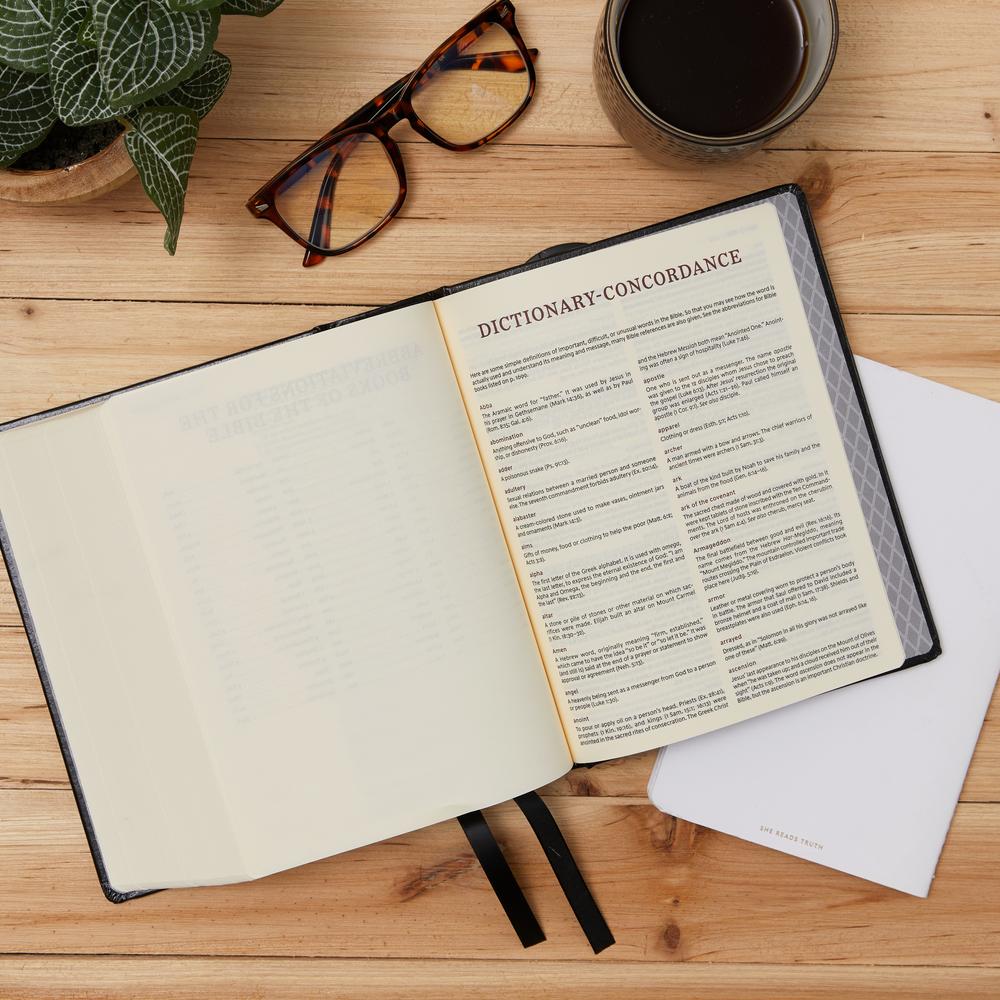The top-down view of this light-colored wood grain desk reveals a meticulous arrangement of items. On the top left, a pair of black and brown reading glasses rests near a potted plant with green leaves adorned with white veins. At the top right, a steaming mug of coffee sits ready for a sip. Dominating the center of the image is an open dictionary, displaying definitions under the heading "Dictionary Concordance" at the top of the page. The right page is filled with text while the left remains blank. Several black felt ribbons serve as built-in bookmarks emerging from the bottom of the dictionary, and an additional white piece of paper lies partially beneath the book on the right side. Nearby, a sleek white tablet occupies the right side of the desk, rounding out this orderly and intellectual workspace.